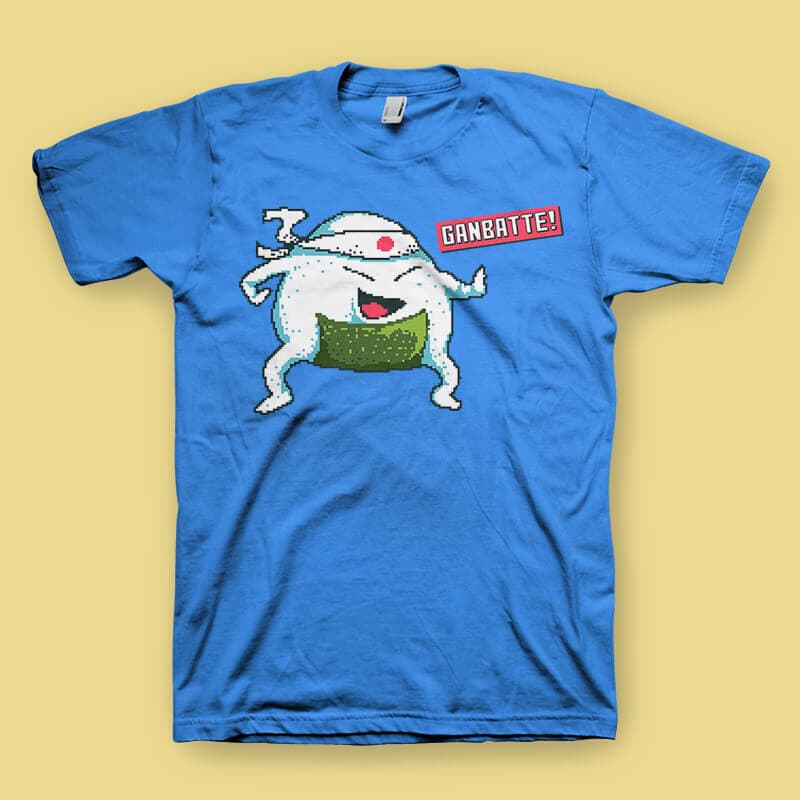This detailed photograph features a cyan-colored, short-sleeved cotton t-shirt spread out on a light yellow table. It is a unisex, child's size shirt with visible wrinkles towards the bottom center and across both the left and right sleeves. The t-shirt prominently displays a cartoon character with a rounded shape similar to a rice ball or egg, and features four limbs—two legs and two arms. The character wears a Japanese-style head wrap or bandana and a green seaweed covering below its mouth. Positioned to the right of the character in a slanted red box is the word "GANBATTE!" in white letters. A white tag is visible at the back of the shirt, further indicating the casual and laid-back nature of this playful design.